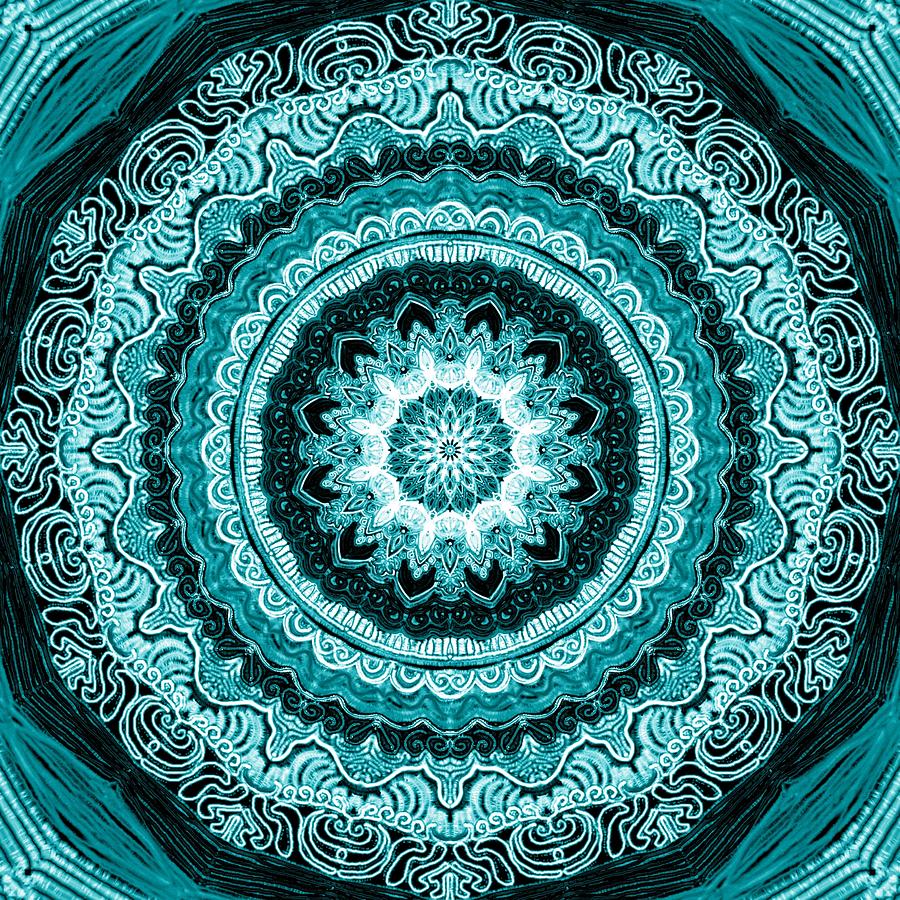This square image resembles a mandala design and appears to be crafted from various fabrics, giving it a tactile, layered depth. It features a harmonious blend of blues—sky blue, turquoise, teal, light blue, and dark blue—along with white. At the center lies a spirograph-like star pattern in white, radiating outwards through multiple concentric circles of intricate design. These circles transition through shades of white, sky blue, teal, dark blue, and incorporate scalloped edges, wavy tile patterns, and ornate rounded filigree-type scrolls towards the outer edge. Each corner of the image is accented with teal and sky blue lines. This pattern is so meticulously detailed that it creates an optical illusion, drawing the eye toward the center, which boasts an even more elaborate lotus flower design. The tapestry-like appearance of the image, with its array of swirls and flower motifs, evokes the sense of a giant, intricately patterned, tie-dye fabric artwork.